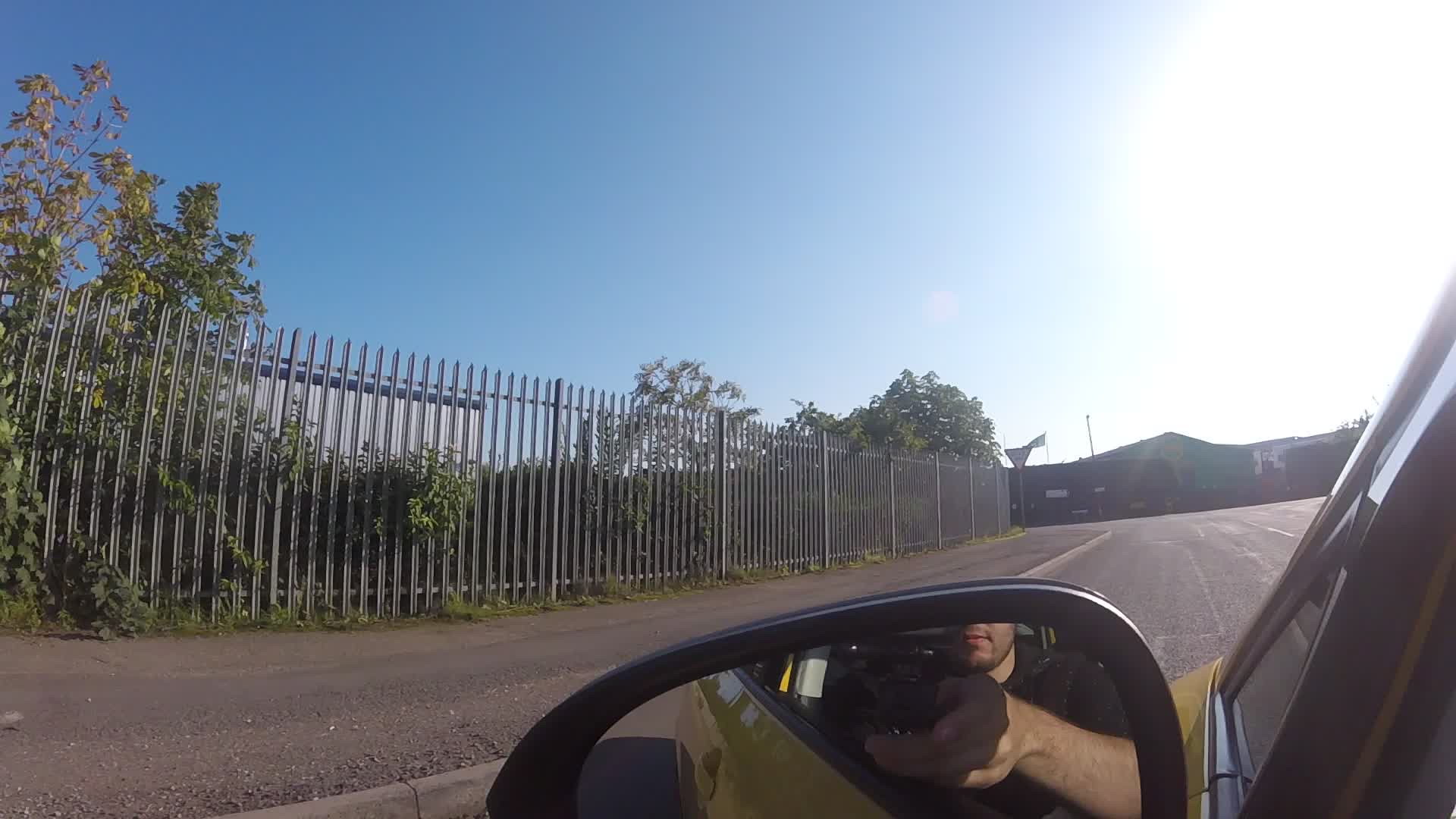A vibrant photo captures a man sitting in a small yellow car, taking a picture with his left hand holding a camera out of the driver's side window. His slightly bearded face and olive-skinned arm, adorned with dark brown to light black hair, are visible in the car’s rear-view mirror. The scene outside the window includes a tall metal fence with trees poking through it on the left side, next to a sidewalk and curb. Ahead of the car, which occupies one lane of the road, are short one-story buildings. To the right of the frame, the rooftops of houses silhouette against a cloudless blue sky, while a giant white blur from the sun occupies the top right corner. The road, which might suggest driving on the left side, further adds to the depth and intrigue of the photograph.